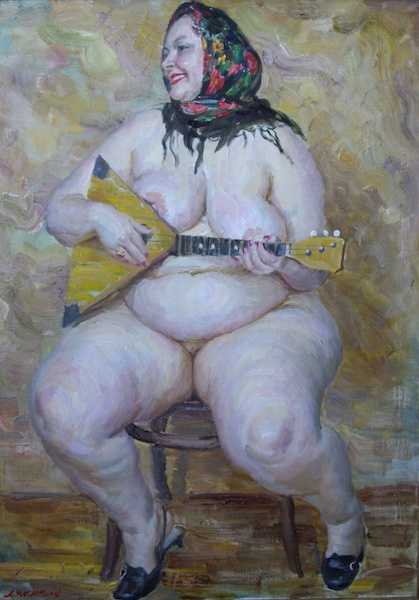This detailed vertical rectangular painting depicts an older, heavyset woman, likely in her late 50s or 60s, sitting on a stool with black shoes featuring buckles. The only article of clothing she wears is a colorful, fringed scarf on her head, decorated with yellow, pink, and green flowers on a black fabric. She has a pale complexion, red lipstick, and a warm smile on her face as she looks to the left. Holding a triangular, light-colored Russian string instrument, she positions her right arm over the triangular part while her left hand rests on the strings, giving the impression she is playing. Her large breasts and stomach are partially obscured by the instrument, and her legs, bent at the knees, rest firmly on the floor. The background features a swirled pattern of grays, browns, beiges, with hints of green, purple, and red, while the floor displays shades of brown, light and dark, mixed with gray, resembling wood.